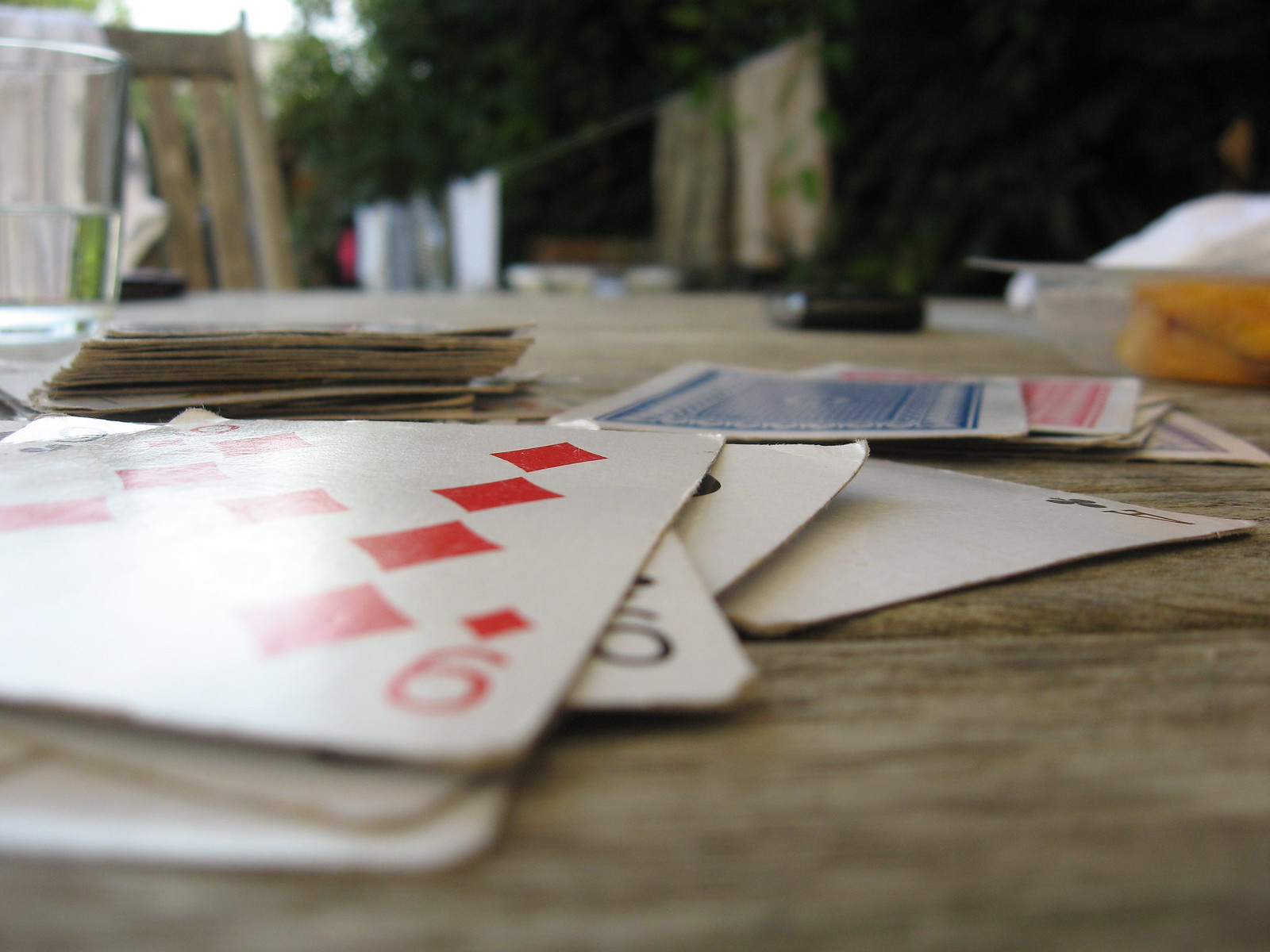This photograph captures a close-up scene of a wooden table, although the focus and angle make the exact material difficult to confirm. The table surface is scattered with playing cards, some face-up and others face-down. The face-up cards prominently display a nine of diamonds and a black nine, with the suit indeterminate between spades or clubs, and an ace of clubs. Additional cards lay partially obscured by these face-up cards, while others exhibit distinctive blue and red patterned backs. Behind these cards, a stack of more playing cards is visible. The blurry background features patches of green, brown, and dark tones, creating an indistinct setting. To the side, there's a plastic container with something orange inside, adding a splash of color to the scene and hinting at a casual, possibly game-related environment.